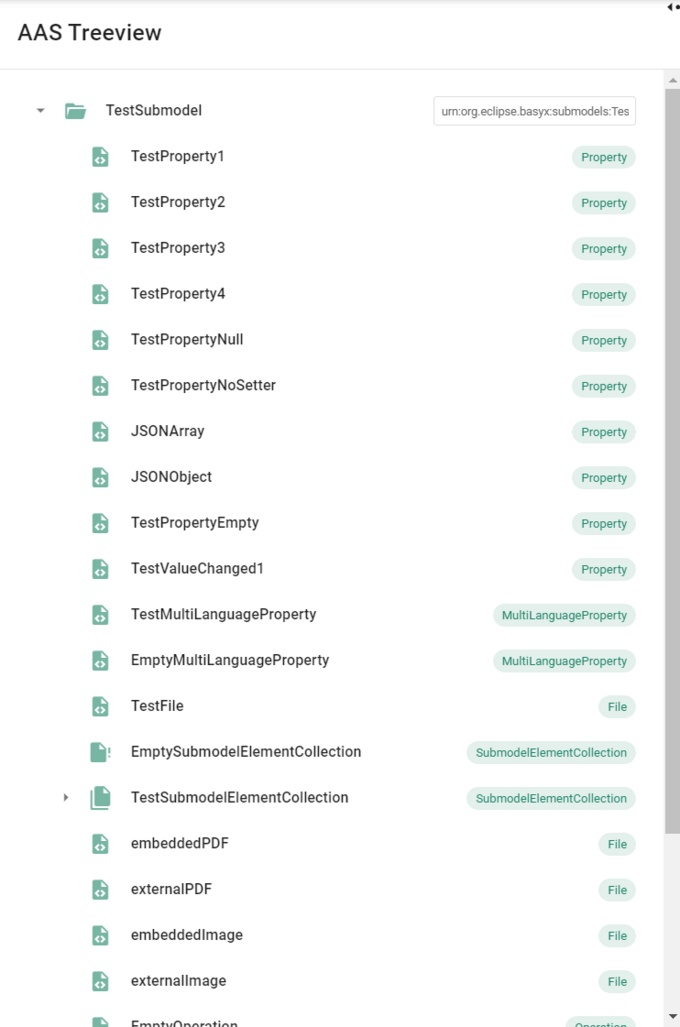The image showcases a computer screen displaying a software interface labeled "AAS TreeView" in prominent black lettering at the top. Directly underneath, there is a black down arrow followed by a green folder icon labeled "Test Submodel". Below this, are a series of green folders with associated labels and descriptions. The first green folder is named "Test Property" with the descriptor "Property" to its right. Subsequent entries include "Test Property 2", "Test Property 3", and "Test Property 4", each labeled "Property" on the right as well. Another folder is labeled "Test Property NULL" with "Property" to the right, followed by "Test Property NULL centered", also described as "Property".

Continuing down the list, there is "JSON Array" and "JSON Object", each with "Property" to their right. The interface also includes a folder labeled "Test ValueChanged 1" with "Property" to the right, and more complex entries like "TestMultiLanguageProperty" and "EmptyMultiLanguageProperty", both distinguished with "MultiLanguageProperty" to the right.

Further down, there are specialized items such as "TestFile" labeled "File" to its right, followed by "EmptySubmodelElementCollection" marked as "SubmodelElementCollection". Finally, the list concludes with specific file designations: "EmbeddedPDFFile", "ExternalIPDFFile", "EmbeddedImageFile", and "ExternalImageFile", all with "File" indicated to their right.